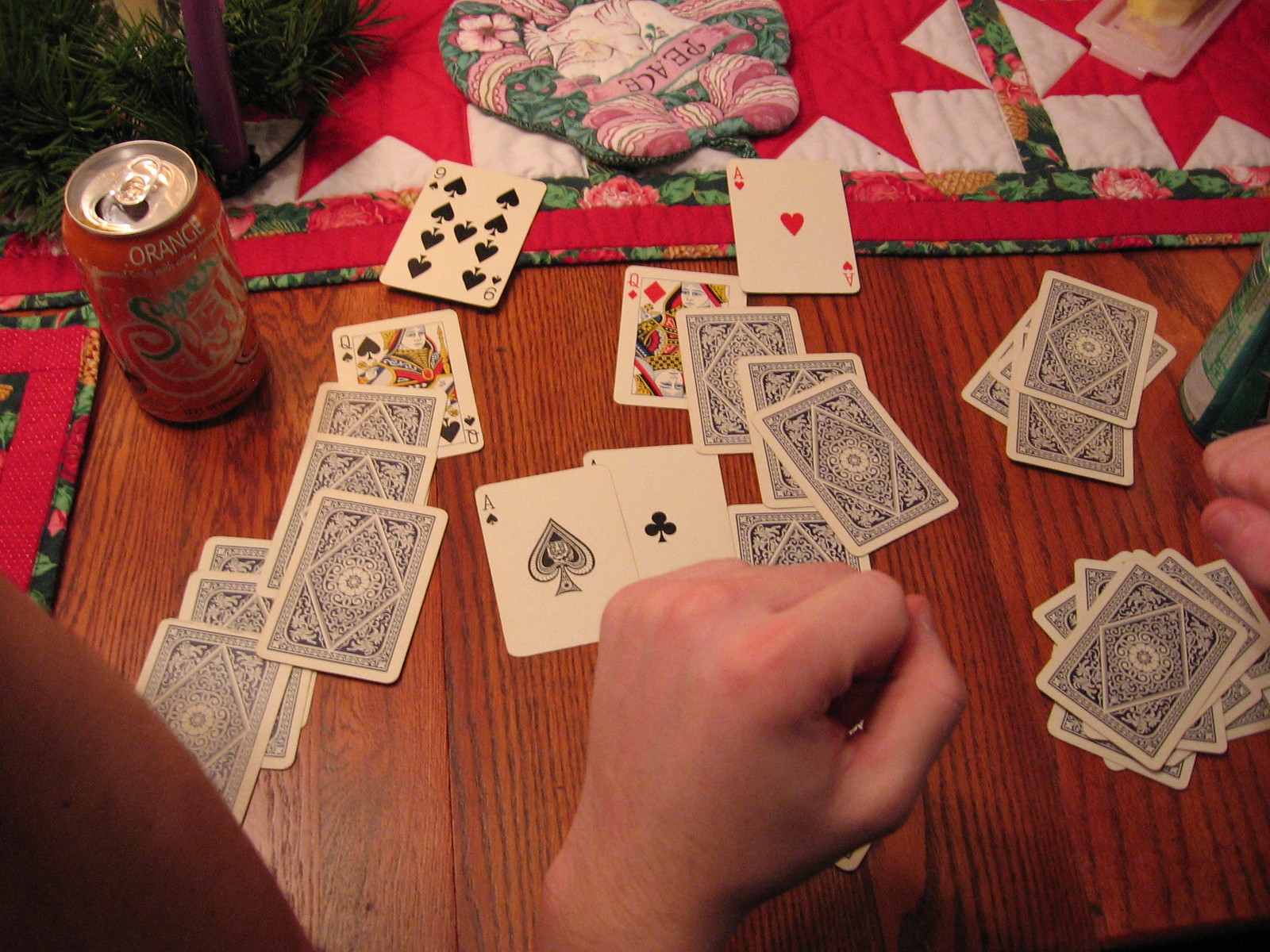This indoor photograph captures an engaging scene centered around a lively game of cards. In the upper left corner, an orange soda can with green lettering stands out, displaying the brand name "Super Chill" in vibrant colors. The table or floor is strewn with playing cards that include a queen of spades, nine of spades, ace of hearts, queen of diamonds, ace of spades, and ace of clubs. A white fist is prominently positioned in the center, suggesting active participation in the game. Additional cards are organized into several piles across the surface. In the upper right corner, another hand is seen, emphasizing the involvement of multiple players. Accompanying the orange soda can is another green soda can, though its label is unreadable. Adding a touch of homeliness to the scene, a quilted, homemade table runner stretches across the middle of the area. It features a red edge, a floral border, white squares, and an attachment with the word "Peace," enhancing the warm, comforting atmosphere of the gathering.